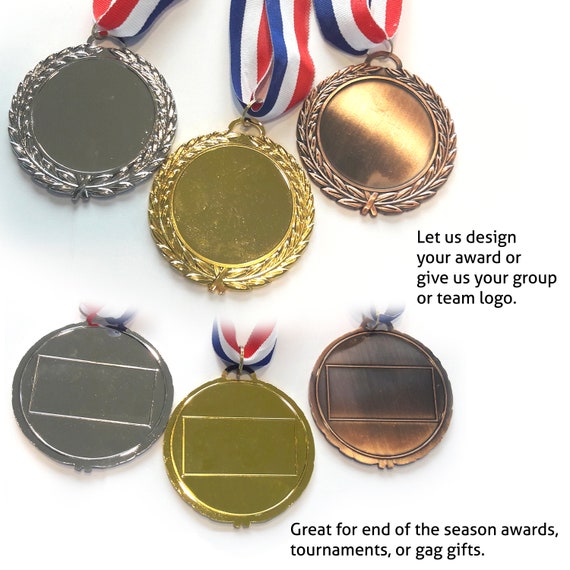This image showcases an advertisement featuring six blank medals designed for customizable awards. The medals are arranged in two rows against a white background. Each medal is attached to a red, white, and blue ribbon reminiscent of an American flag. 

The top row displays gold, silver, and bronze medals, each with a decorative floral-leaf arrangement around their borders. A small portion of their ribbons is visible. The bottom row also has gold, silver, and bronze medals, but these feature a simpler beveled edge design with an engraved rectangular area for personalization. The ribbons are less visible here.

Both rows of medals are accompanied by black text. Above the top row, it reads, "Let us design your award or give us your group or team logo," while below the bottom row, it states, "Great for end of the season awards, tournaments, or gag gifts." This promotional image demonstrates how the medals can be customized with logos or text to suit various occasions.